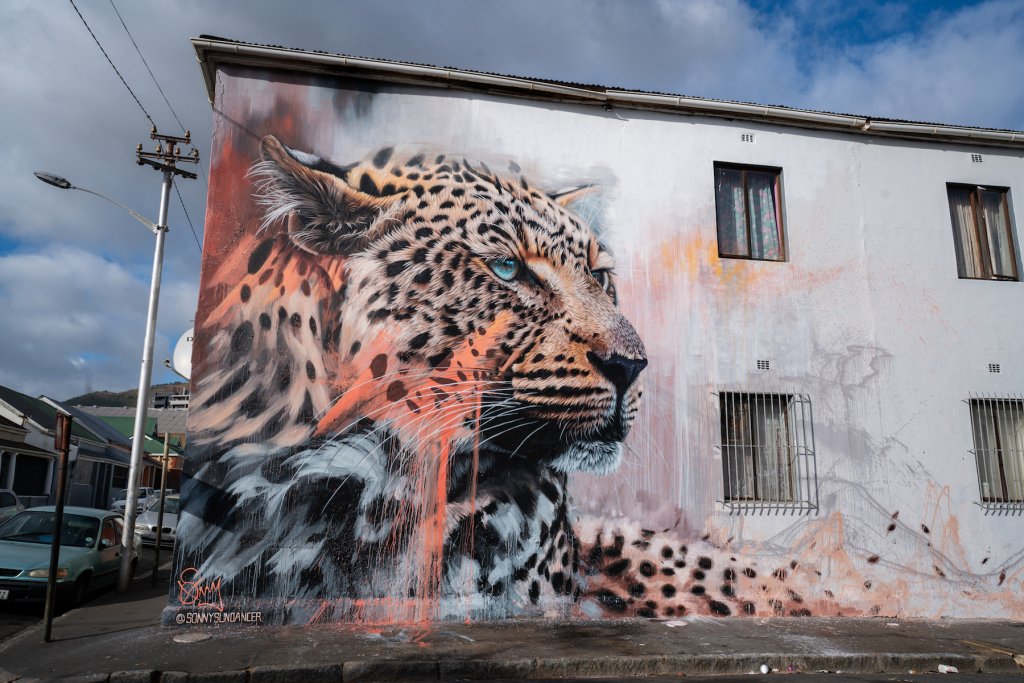The image features a striking mural of a cheetah with vibrant turquoise eyes and dark spots, painted on the corner of a two-story building with a flat roof. The cheetah, depicted with a serious and alert facial expression, showcases its readiness to spring into action. Bright teal eyes stare wide open, enhancing its intense demeanor. The mural includes orange paint streaks dripping down the cheetah’s face, creating a dramatic effect. 

The white wall of the building hosts four windows with bars on the lower ones, suggesting a rougher neighborhood. A dark gray sidewalk runs in front of the building, beside which cars are parked along the street. In the background, the sky is filled with white clouds, and a streetlight pole is visible to the left. The mural, situated prominently on the left corner of the building, is signed "Sunny Sun Dancer" at the bottom.